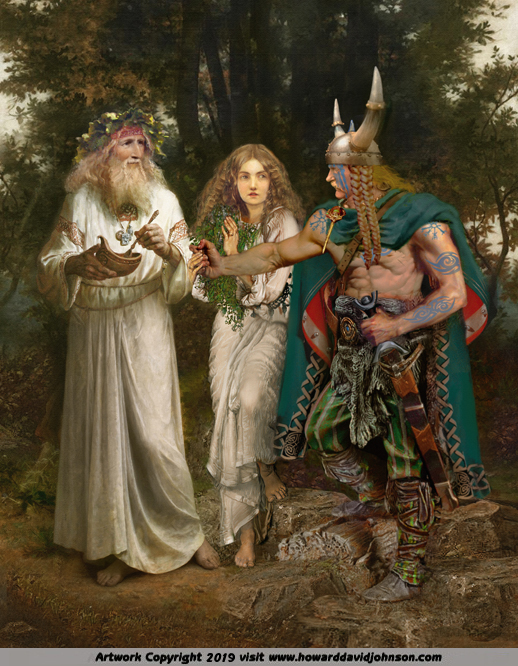In a vertical, art print-style image set outdoors among trees, a shirtless, muscular Viking with long braids, adorned in blue rune tattoos and wearing a gold, two-horned helmet with chains, stands prominently. He sports green striped pants and a green rope over his shoulder, with one hand resting on a sheathed sword. The Viking gazes intently at a serene, angelic-looking couple dressed in long white robes. The older man, with a long beard, holds a mysterious object in his hand while the young woman beside him stands innocently. Both are barefoot, exuding an aura of purity. At the bottom, the image is captioned with "artwork copyright 2019 visit www.howarddavidjohnson.com."